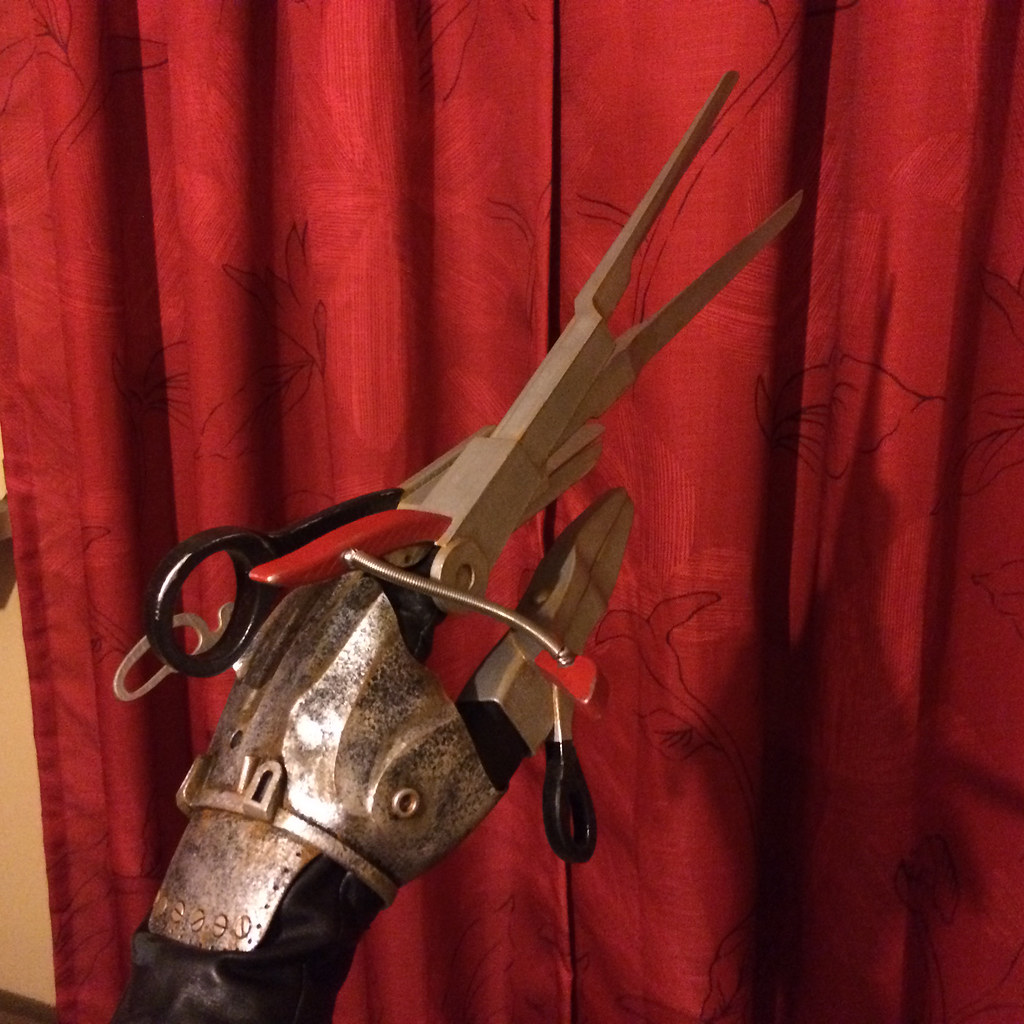The photograph features a detailed image of a robotic left hand emerging from the bottom left corner, set against a backdrop of red, floral-patterned curtains with a small section of a light brown wall to the side. The hand, which resembles a simplified version of the iconic Edward Scissorhands glove, showcases a metallic armor-like construction. The fingers of the hand are particularly striking: the pointer finger is squared off with a blade at the end, and the middle finger mimics the appearance of one blade from a pair of scissors, complete with a black handle extending above the knuckles. The thumb features a pull rod with a black loop. The overall structure includes silver piping and appears to be a functional tool prototype, possibly a wearable scissors glove, with red and black adjustment handles and loops visible.